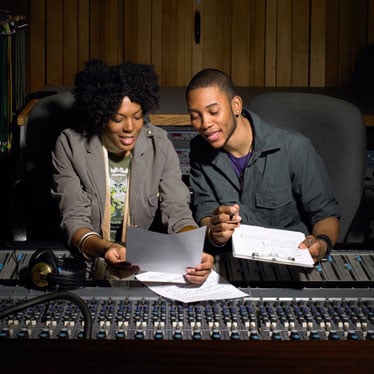In a dimly lit recording studio with wood-paneled walls, a man and a woman are intently collaborating over a large audio soundboard. Both of them are seated in office chairs, with their forearms resting on the board. The man, positioned on the right, holds a clipboard, while the woman on the left holds a loose sheet of paper. They are both focused on the sheet in the woman's hands, smiling and discussing its contents. A pair of headphones lies to the left of the woman, adding to the ambiance of a music production session. The overall scene is accented with shades of brown, gray, blue, white, and black, though the specific time of day remains indeterminate. It is clear they are deeply engaged in reviewing and improving their music, making sure the next song is the best it can be.